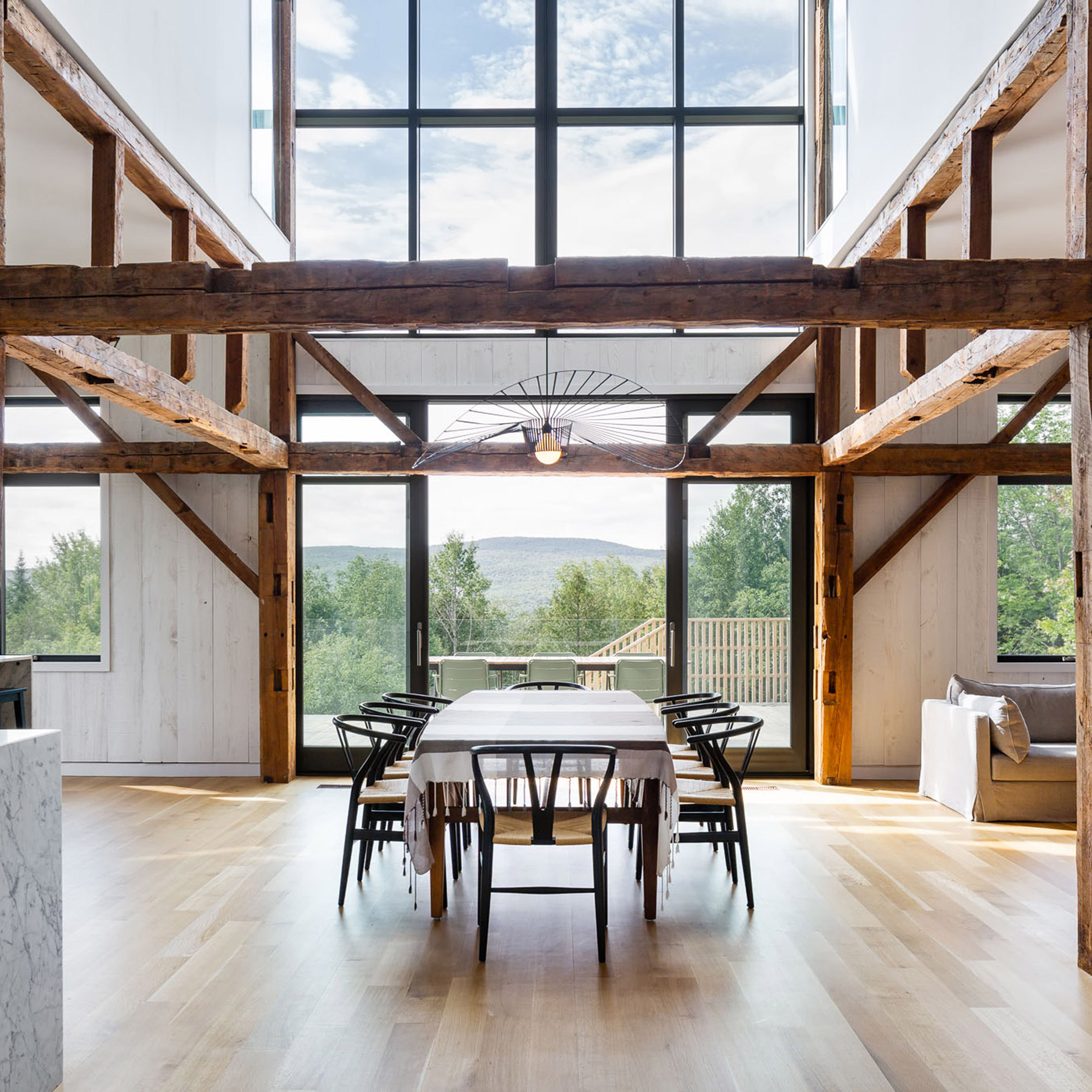This detailed photograph captures the essence of a beautifully designed dining room with a striking view of nature. The spacious interior features pale hardwood flooring that spans the lower third of the image, complemented by a grey canvas couch on the far right and a glimpse of a marble counter at the frame's edge on the left. The walls are adorned with painted white vertical wood panels, accented by natural stained wood square supports that flank a set of two black-framed glass doors in the center, topped with a large window. Above these doors is another row of windows that extends upward, providing an expansive, two-story panoramic view of the lush, green forested hills outside. The architectural wooden beams crisscross just below the upper windows, enhancing the room's rustic, yet elegant cabin-like charm.

In the center of the room, aligning perfectly with the central window, stands a rectangular table draped with a white and gray striped tablecloth. The table is surrounded by black metal chairs with wooden seats—one at each end and three along each long side. Above the table hangs an artistic lamp, resembling a swirly, lightweight sculpture, adding a contemporary touch to the rustic setting. The inviting ambiance of this dining room blends seamlessly with the vibrant greenery visible through the glass doors and windows, making it an idyllic spot for enjoying meals while basking in the scenic outdoor view.